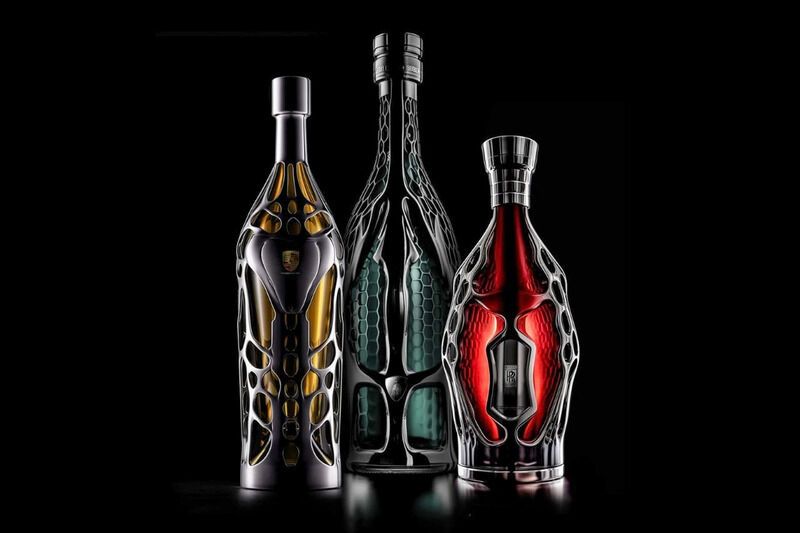This is a highly detailed AI-created image depicting three ornate bottles set against a solid black background, which occupies the majority of the space, creating a stark contrast. The bottles are intricately designed with dark, black or slate-gray armor-like exteriors that appear to be illuminated by an external source. Each bottle features dark-colored caps and reveals vibrant interior colors through openings in their armored shells. The bottle on the left has a yellowish hue inside, the taller middle bottle contains a turquoise green hue, and the shorter, wider bottle on the right displays a radiant red core. The unique characteristics and variations in design across the bottles contribute to an intriguing and visually striking composition.